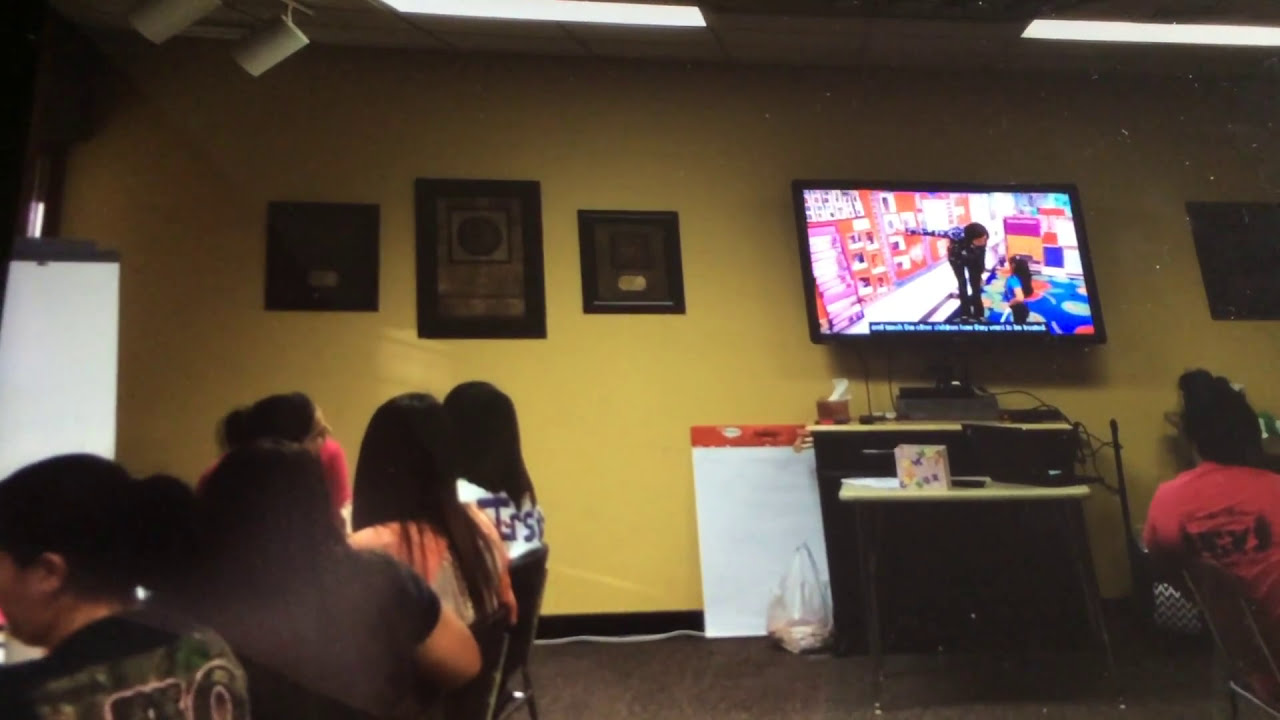This photograph captures a room with a yellow-walled interior, featuring a large flat-screen TV mounted on the right side of the wall. The TV is displaying a children's program where a person appears to be engaging with a child. Situated below the TV, there is a black stand with a yellow top, and next to it on the ground, is a white object. In the foreground on the left, multiple people—mostly women with long hair in casual t-shirts—are seated on chairs facing the television. Behind these chairs and toward the center of the wall, three photographs or paintings and several boards or plaques are prominently displayed. There is also a person in a red shirt with black lettering seated to the far right, also engrossed in the TV program. The room is dimly lit, with fluorescent light fixtures and spotlights visible on the ceiling, although these lights are turned off. Several tables with various items are also seen across the room.